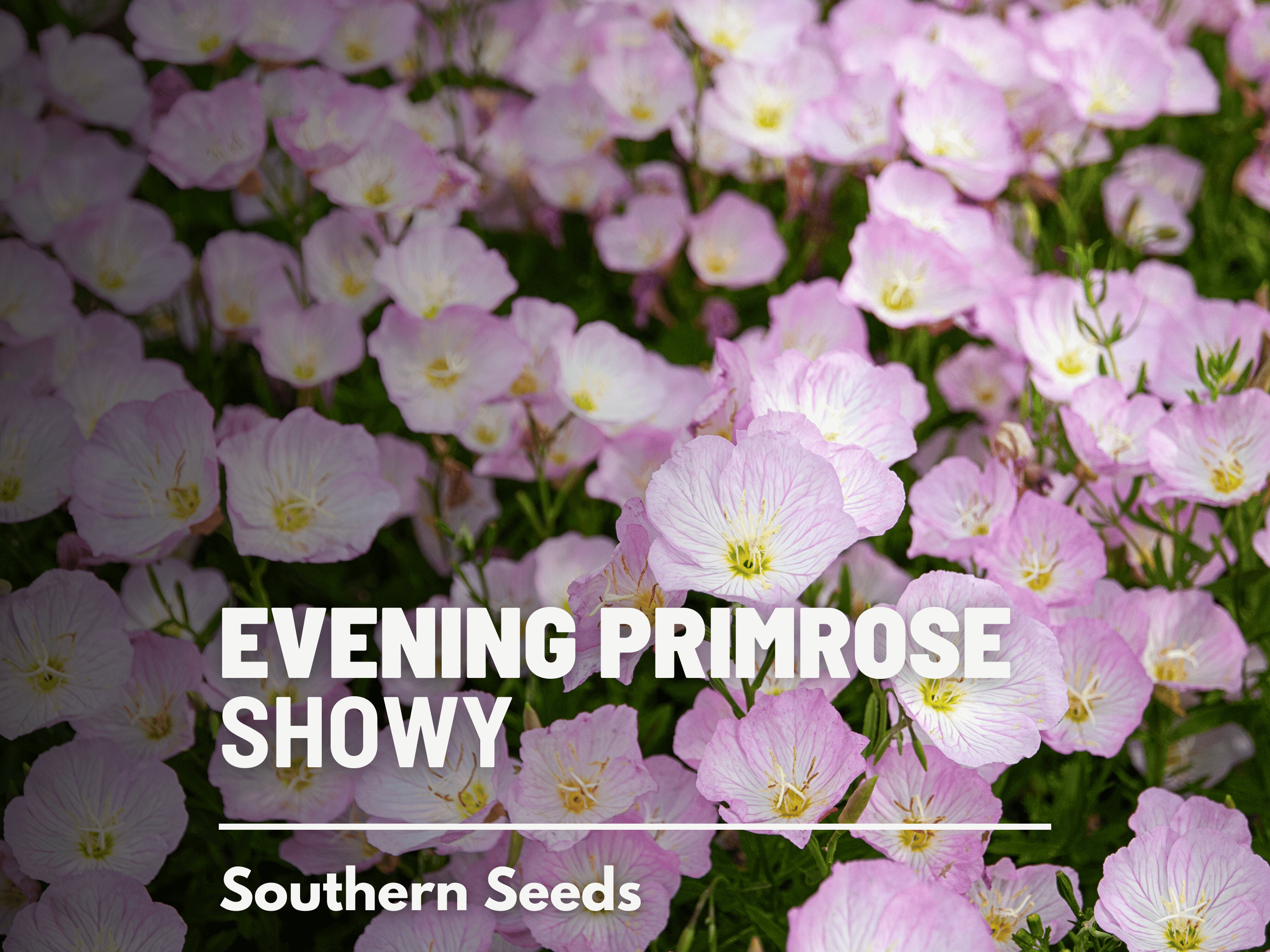The promotional image features a picturesque field of Evening Primrose 'Showy' flowers in full bloom, showcasing a stunning display of delicate flowers with a pinkish-white hue, subtly accented by lavender and white tints. Each bloom has a distinctive yellow-green center, contrasting beautifully with their lush green bases and surrounding foliage. The composition draws the eye to a focused area in the lower right-hand corner, while the rest of the image has a softly blurred background, adding depth to the floral scene. Dominating the bottom of the image, bold white text reads "EVENING PRIMROSE SHOWY" followed by a white horizontal bar and "SOUTHERN SEEDS" in all caps, indicating that this is likely a seed packet cover illustrating what the flowers look like when in full bloom. This captivating visual captures the essence and allure of Evening Primrose 'Showy' from Southern Seeds.